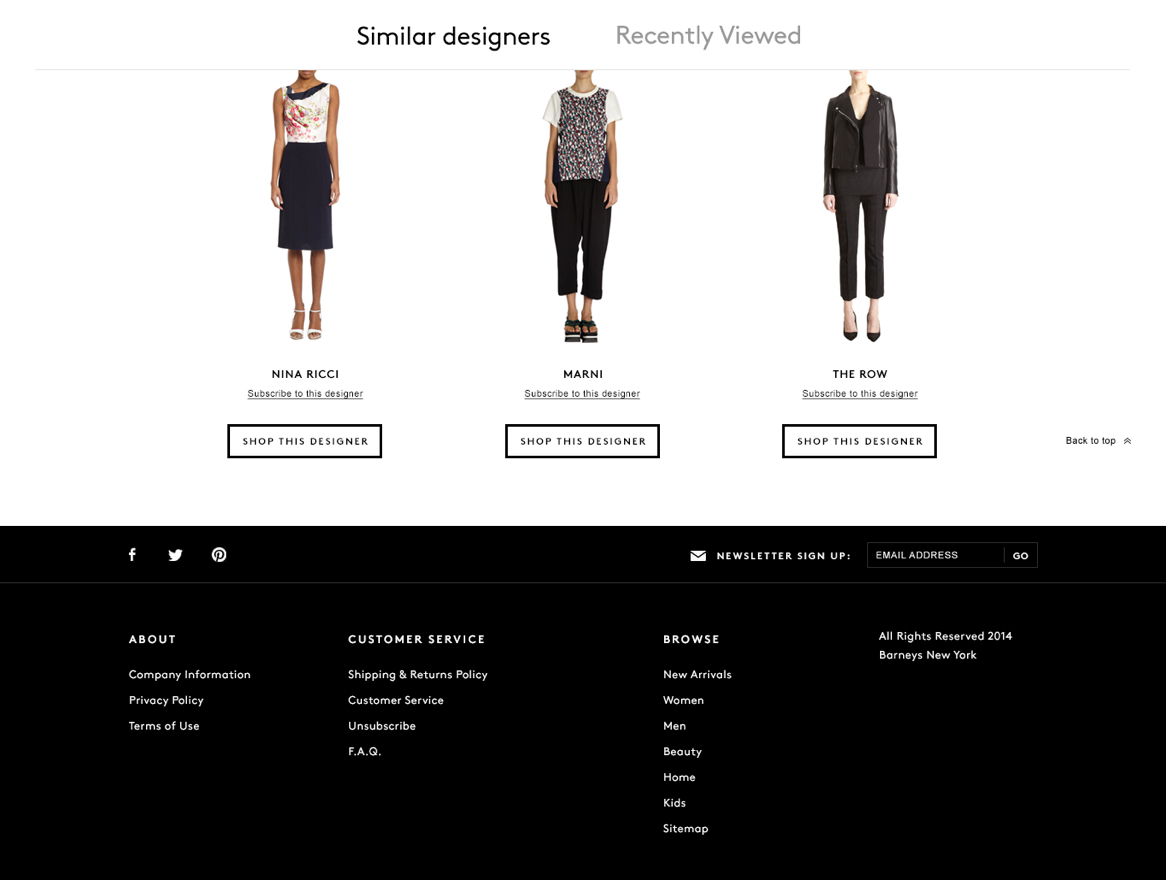The screenshot displays a section from a website's interface featuring several interactive options and links. At the top, there are two prominent buttons: "Similar Designs" on the left and "Recently Viewed" on the right. Below this, three designer models are showcased. The first model on the left is labeled "Nina Risi" with options to "Subscribe to this designer" and a button to "Shop this designer." The central model is named "Marni," also accompanied by subscription and shopping options. The final model on the right, titled "The Row," includes similar actions for subscription and shopping.

On the far right of this section, there's a button labeled "Back to the top." The screenshot's lower portion features social media icons for Facebook, the old Twitter symbol, and Pinterest. To the right, there's a "Newsletter Sign Up" prompt with a text box for entering an email address. The footer contains various informational links: an "About" section with company information, privacy policy, terms of use, and customer service details including shipping and returns policy, customer service contact, an unsubscribe option, and an FAQ page. The "Browse" section offers categories such as new arrivals, women, men, beauty, home, kids, and a site map. The screenshot concludes with "All rights reserved, 2014, Barneys New York."